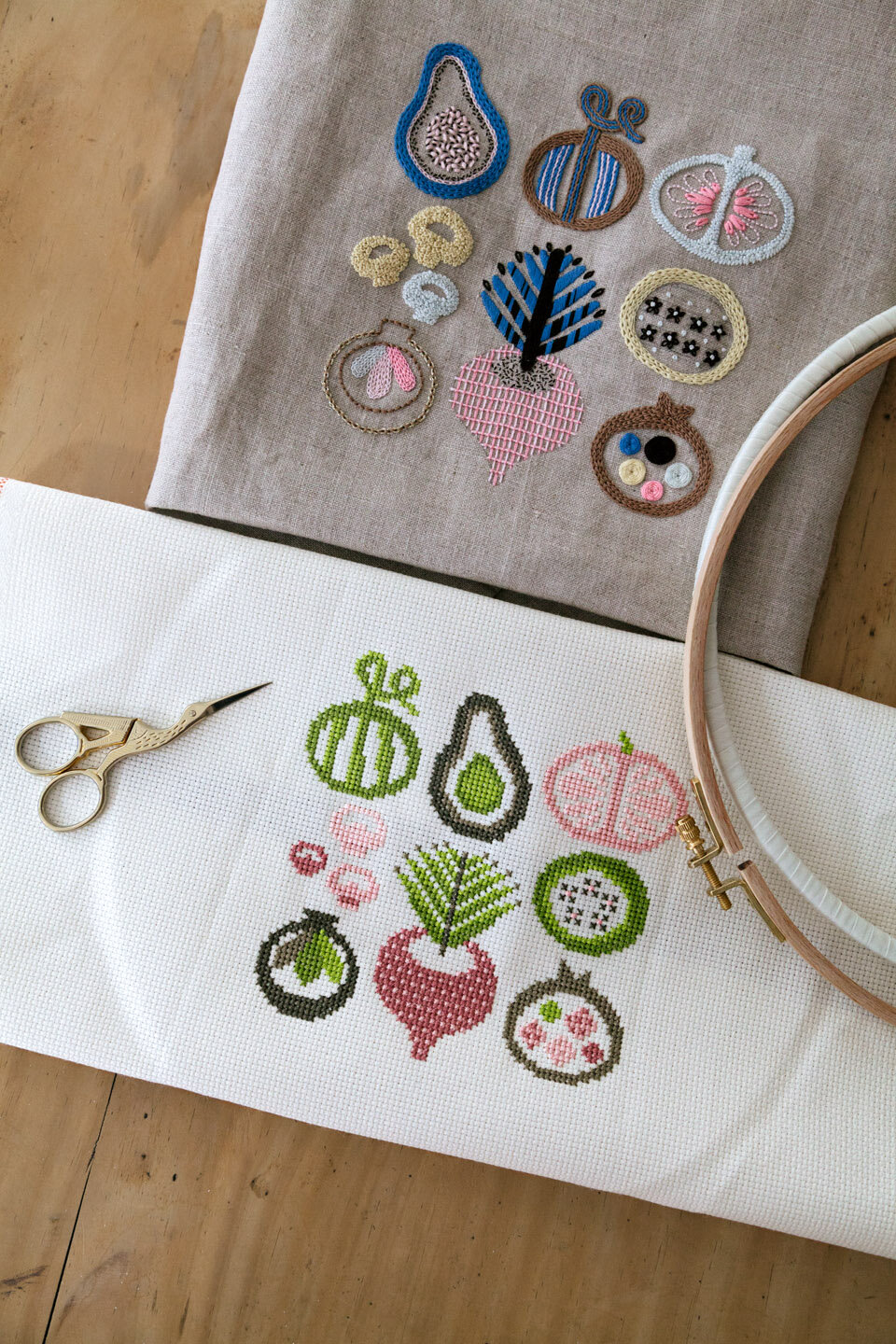The image depicts an intricate embroidery setup taken from a top-down angle. On a rustic brown wooden surface, there are two pieces of fabric showcasing different stages of embroidery. The top fabric, resembling light gray burlap, features vividly colored, minimalist designs of various fruits and vegetables, including pear-shaped objects, apples, and radishes, stitched in shades of blue, pink, and black. Below it, a white fabric is stretched inside an adjustable wooden embroidery hoop, adorned with a similar assortment of embroidered objects like avocados, beets, and grapefruit in colors like green, brown, pink, and red. To the left of the hoop, a pair of small, gold bird-shaped scissors, polished and detailed, lies ready for fine thread cutting. The entire setup exudes a DIY ambiance, highlighting the care and artistry involved in embroidery, juxtaposed against the warmth of the wooden table.